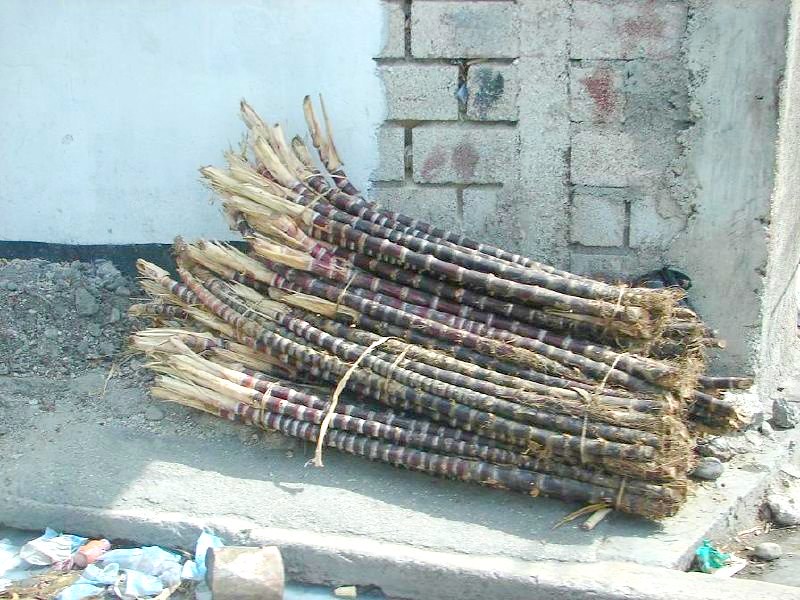The photograph depicts a series of bundled sticks, potentially sugar canes or similar long canes, neatly arranged on a concrete floor amidst scattered debris and dirt. Each stick is dark brown with light brown or beige horizontal stripes and appears to have been deliberately broken by hand to approximately the same length, leaving the ends fuzzy and shredded. The scene is illuminated by clear sunlight, adding to the vividness of the textures. In the foreground, on the left, there is blue and white paper alongside a can and an overexposed orange object, while a green paper is crumpled up in the lower right corner. Surrounding the bundles of sticks are several rocks and more debris. The background showcases a partially painted white wall with black trim on the left side, transitioning into exposed brick and concrete on the right.